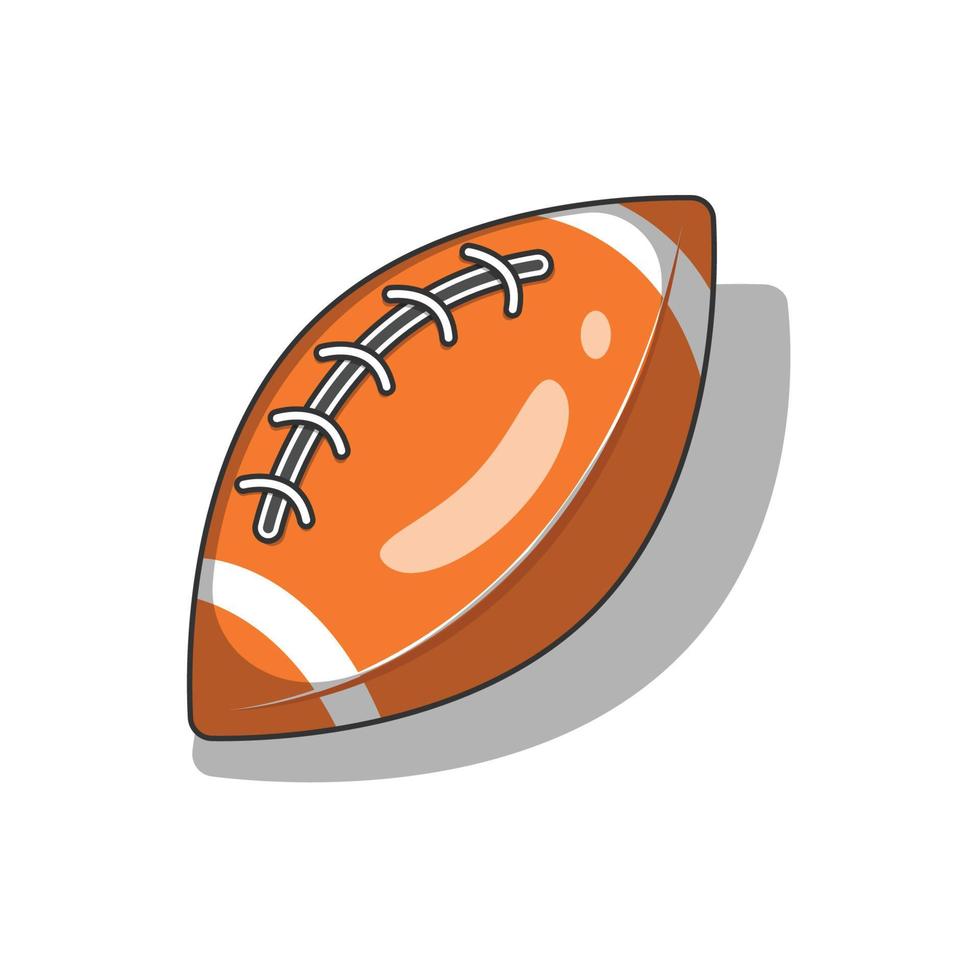This image features a cartoon-like depiction of a football, rendered in a simplistic, animated style with a 3D effect. Positioned at a slant about 30 degrees to the right, the football exhibits a smooth, oval-like shape accentuated by thick outlines. Its surface is a light brownish or orangey-brown color, highlighted by minimal shading and lighting effects that suggest a light source, casting a gray shadow on the white background. The football is detailed with a black arch on top and central white laces, accompanied by two white stripes near each end. The overall aesthetic resembles that of a children's picture book or a sticker, emphasizing its non-realistic, cartoonish appearance.